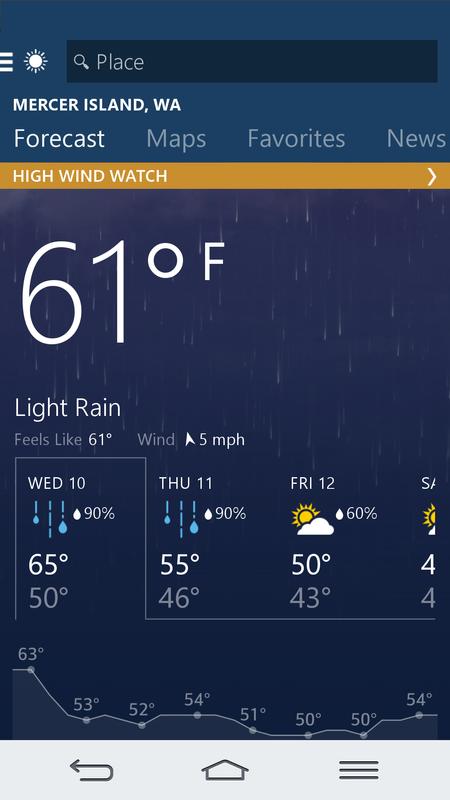This image showcases a screenshot of a weather app on a smartphone. The interface features several elements arranged neatly for easy navigation and information access. 

Starting from the top, there is a hamburger menu located on the left side of the screen next to a sun icon, which stands out against the blue background. Adjacent to this is a search field with a magnifying glass icon on the left, and the placeholder text "Place" inside the field.

Directly beneath the search bar, the location is specified as "Mercer Island, WA." Following this, there are four tabs labeled "Forecast," "Maps," "Favorites," and "News." The "Forecast" tab is currently selected, indicated by its lighter color and a yellow underline.

The primary focus of the screen is the weather alert displayed prominently in white text on a blue background: "High Wind Watch" with an arrow pointing right for more details.

Below this alert, the current temperature is shown in a large font: "61°F." The background here simulates a rainy scene with streaking raindrops. Supporting details include the text "Light Rain," "Feels like 61°F," and "Wind: 5 mph," with the wind direction vaguely northwest.

The forecast extends into the week ahead, with each day represented with line graphics and segmented bars illustrating temperature variations. The detailed forecast for Wednesday, the 10th, is highlighted, showing a 90% chance of rain with a high of 65°F and a low of 50°F. Thursday follows with similar predictions, 55°F high and 46°F low. Friday indicates partly cloudy conditions with a 60% chance of rain, highs of 50°F and lows of 43°F.

Towards the bottom, there is a line graph displaying temperature changes over time, with temperature markers at 63, 53, 52, 54, 51, 50, 50, and 54°F.

Finally, the navigation menu is located at the bottom of the screenshot, offering quick access to other sections of the app.